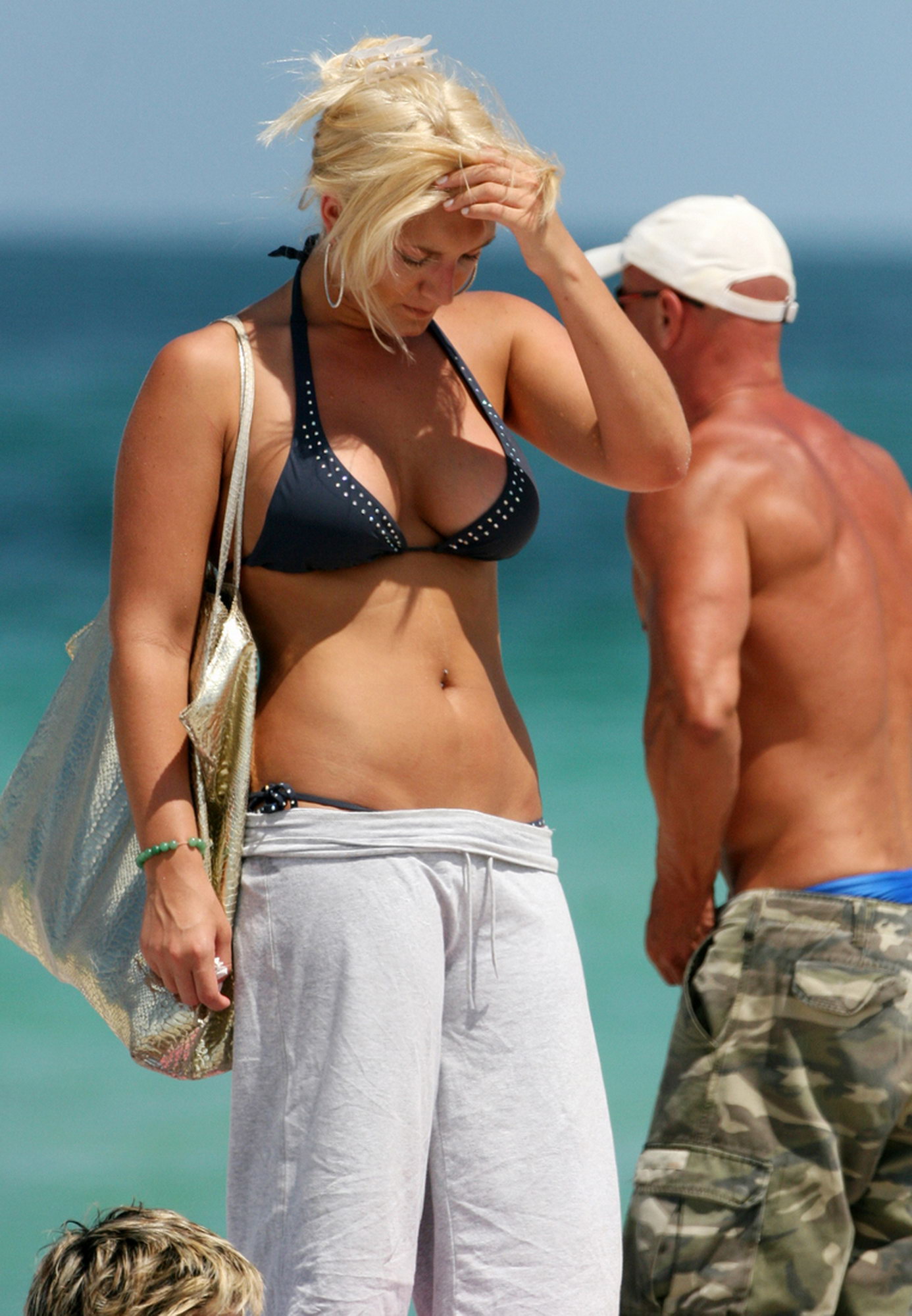This image captures a bright, sunny day at the beach, featuring a central pair of a tall, long-haired woman and a shirtless man. The woman, positioned slightly facing the camera, wears a dark bikini top and whitish sweatpants, with a large white purse slung over her right shoulder. Standing to her left, the man sports a white hat and camouflage cargo shorts, with blue-rimmed underwear visible underneath. In the bottom left of the image, the top of a young boy’s blonde head emerges. The backdrop showcases a vast, serene body of water under a light blue sky, and the sandy beach extends beneath the feet of the subjects. The colors in the image include varied shades of blue, tan, green, and white, and there is no text present. This outdoor scene exudes a relaxed, daytime beach atmosphere.